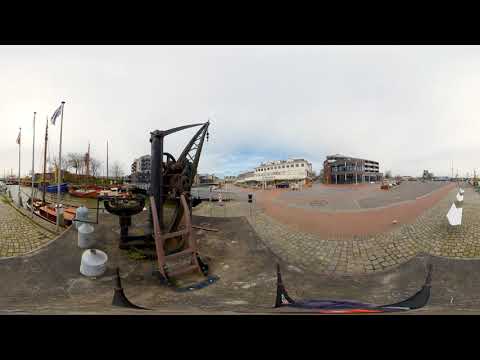This rectangular photograph, bordered by black bars on the top and bottom, captures an expansive outdoor scene dominated by a massive white cloud with a small patch of blue sky. The image portrays a slightly distorted panorama where several elements are evident. 

In the foreground on the right, there is a dirt road that curves towards the viewer, flanked by cobblestone walkways. Adjacent to the road, on the bottom left, lies a rusted metal structure resembling an old crane or antique machinery, possibly reminiscent of farm equipment. Surrounding this structure are several flagpoles, some bearing listless flags, stretching vertically towards the sky. 

To the left of the crane, the photograph reveals what looks like rusted steps leading up to more outdated equipment. In the background, the scene becomes more detailed with an array of tall buildings. A significant white building, potentially with multiple stories and viewing areas, stands prominently. Beside it, to the right, a darker, partially constructed or open-framework building can be seen. The dirt road, bordered by cobblestone and a guardrail, arcs through the area, guiding the eye towards the midground and blending into the overall worn but intricate landscape. The distant buildings feature multiple windows and doors, adding an additional layer of depth to this complex, nostalgic scene.